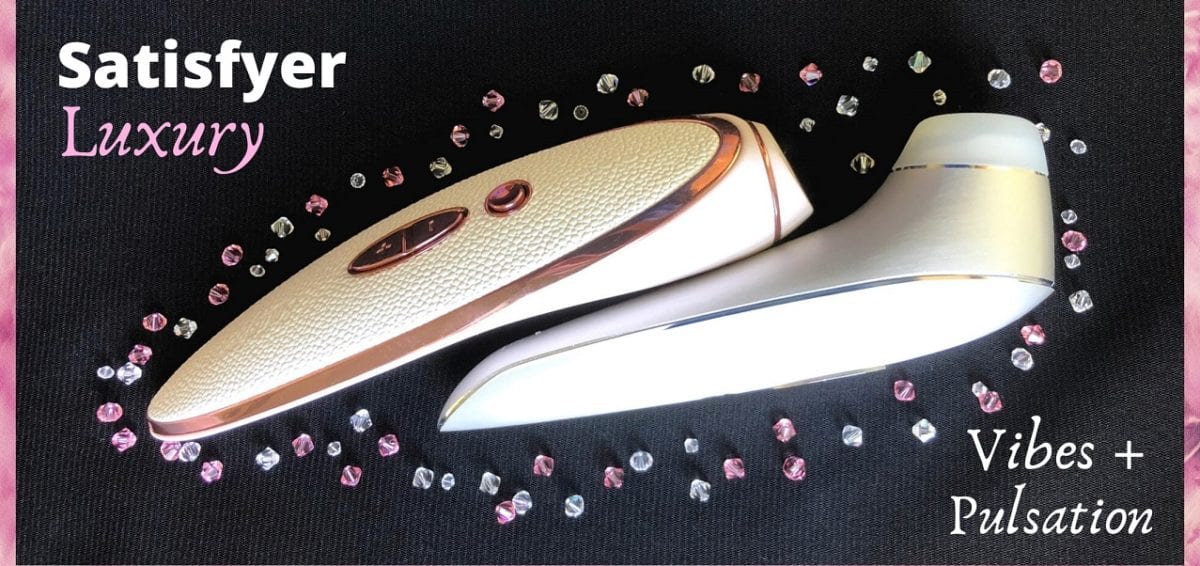This image is a meticulously arranged product advertisement, likely for sale on an adult product website. The rectangular image features a thin purple border on the left and right sides, framing a textured dark grey or black background that appears to have a material-like finish. 

In the upper left corner, bold white text reads "Satisfyer," with "Luxury" elegantly written in purple underneath. Positioned centrally in the image are two identical white and rose gold items, displayed from different angles to showcase their design features. One of the units, oriented in the top center sweeping down to the left, has an oval gold button in the middle and a round gold button beside it, highlighted by a rose gold outline around the top, giving off a leather-like appearance. 

The second unit on the right, angled similarly from the top right down to the left, has three distinct sections: a light clear colored top, a metallic silver middle, and a white bottom. Both units seem to be adult vibrators, indicated by the suggestive placement and detailing.

Surrounding these two objects are light pink and clear crystals of varying sizes, resembling beads due to visible channels through their centers, which enhance the luxurious presentation. In the bottom right corner of the image, "Vibes + Pulsation" is prominently displayed in white text, solidifying the impression that this product is intended for adult use and marketed towards those seeking pleasure-inducing items.